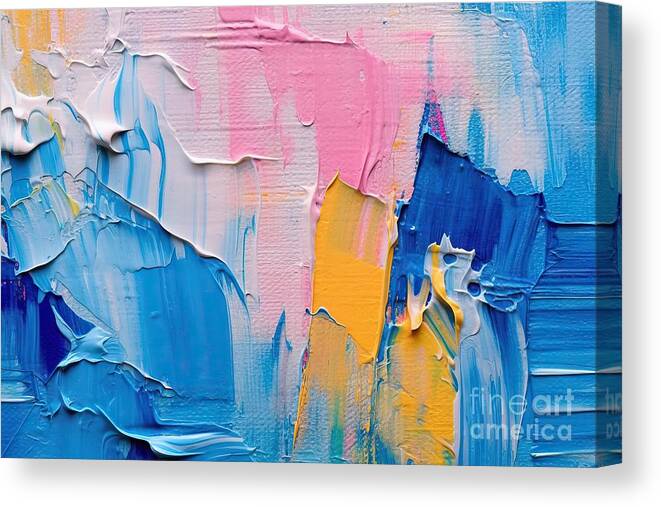The image depicts an abstract painting, possibly displayed on a wall or laid on a white surface, with the text "Fine Art America" inscribed in the bottom right corner. The painting features a variety of colors including light blue, regular blue, dark blue, shades of gold and yellow, pink, light pink, orange, white, and black. The composition shows a pronounced use of textures, giving the surface a rough and uneven appearance with areas of paint thicker in some spots. Gold is predominantly centered, with light and dark blue hues at the bottom left and far right. Pinks are mainly situated near the top. The photograph was taken from a side angle, providing a unique perspective on the artwork. The colors and textures suggest no particular subject but rather an expressive and dynamic assortment of brush strokes and compounded elements, creating a visually engaging abstract piece.